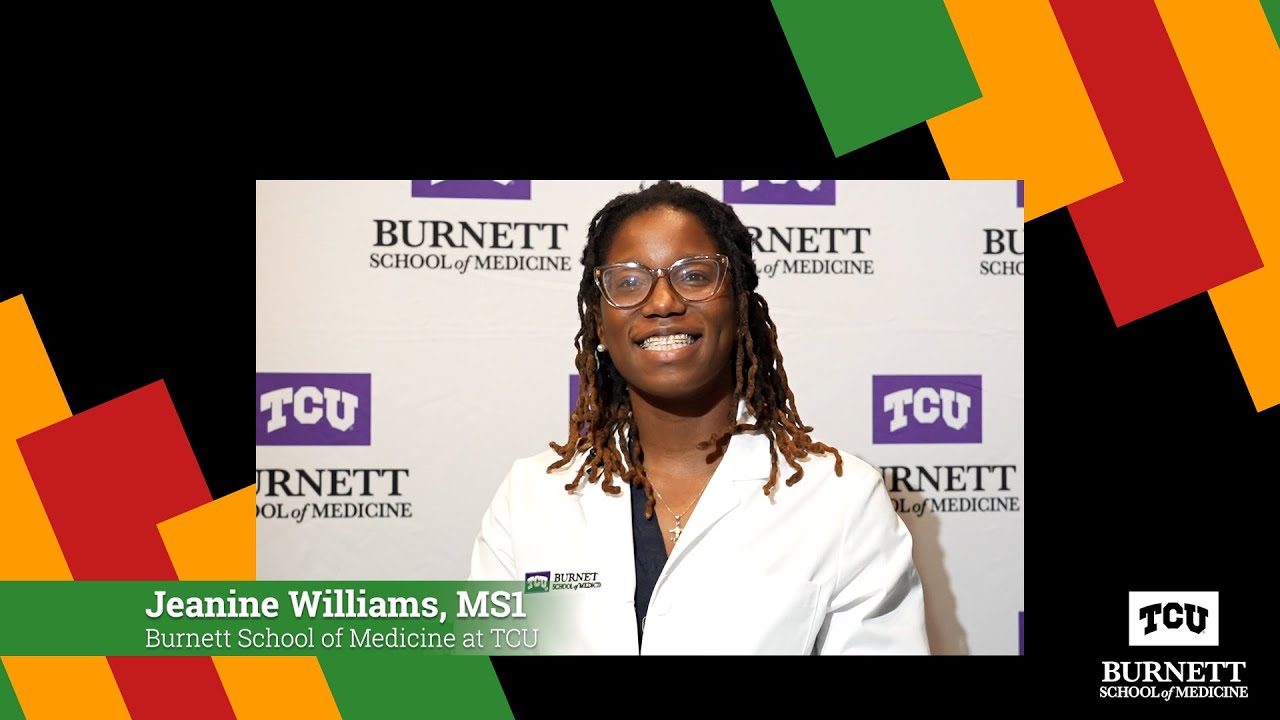This photograph, set in a landscape orientation within a colorfully illustrated landscape background, features Janine Williams, MSI, of the Burnett School of Medicine at TCU. An African American woman with shoulder-length braided or dreaded hair, dark at the roots and lighter at the tips, Janine is captured smiling and gazing up at the viewer through cat-eye glasses. She is depicted from the top of her head to mid-chest, wearing a white lab coat over a darker shirt. Behind her is a banner wall adorned with the TCU logo in bold white letters, and below it, the text "Burnett School of Medicine" in black. The entire photograph is inset into a black background. Artistic, angled shapes in green, yellow, and red decorate the top right and bottom left corners, creating a dynamic visual contrast. At the lower right corner, the TCU logo is prominently displayed. A green horizontal band across the bottom left of the photograph reads "Janine Williams, MSI" in white text, followed by "Burnett School of Medicine at TCU."